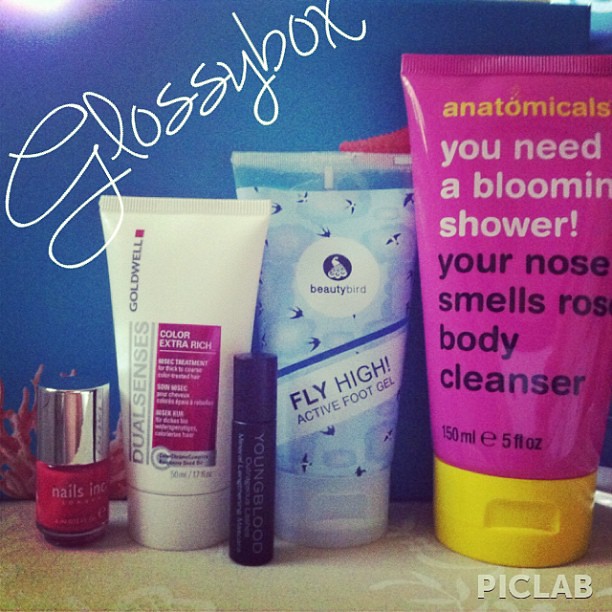The image showcases a selection of cosmetic bottles and tubes against a blue background, with thin, handwritten text at the top reading "Glossy Box" in white. The packaging box, visible at the top and partially masked by one of the products, features some graphics in the bottom right corner.

From left to right, the smallest item is a cylindrical glass bottle with a large silver cap, containing red and pink liquid, labeled "Nails Inc" in white text. Adjacent to it is a thin white tube marked "Goldwell Jewelness, Color Extra Rich" within a pink rectangle.

Centrally positioned between two tubes, there's a tall, thin cylinder with the brand "Youngblood" on it, rendered in purple with black accents. To its right is a sealed tube designed with a blue background and black bird outlines. It carries a circle in the center reading "Beauty Bird" and a diagonal white banner saying "Fly High, Active Foot Gel."

On the far right is a large pink tube emblazoned with the text "anatomicals" in yellow. Below this, in white, it states "You Need a Blooming Shower," and further down, in black, "Your Nose Smells Rose, Body Cleanser, 150 ml E5FL-OZ." The tube is completed with a yellow cap. At the bottom of the image, in capital letters, is the text "Pictolab."

Overall, this detailed composition suggests a curated collection of beauty products, likely part of a promotional Glossy Box, designed for various skincare and beauty routines.